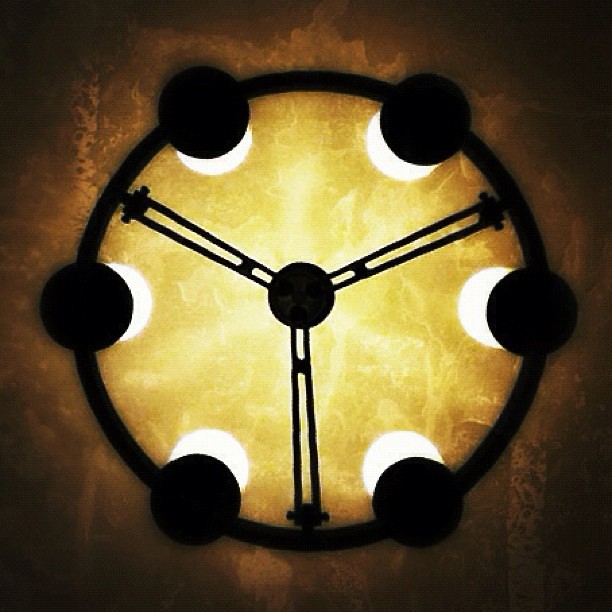This photograph depicts a captivating piece that straddles the line between a functional clock and elaborate artwork. The centerpiece is a black metal ring forming a perfectly round frame. Positioned equidistantly around the exterior of this metal ring are six black circles, each serving as a source of light that emits a soft, glowing luminescence. Intriguingly, the central part of the piece features a black circle from which three slender arms radiate outward, connecting to the outer ring. The entire structure is bathed in a subtle glow, further enhanced by the illumination beneath the black circles. The radiant artwork is set against a textured background with a rustic brown hue, adding an earthy and aged aesthetic to the overall composition.